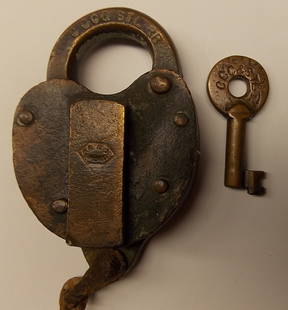The photograph depicts a very old and antique lock and key, set against a light brown beige background. The background is uniformly colored, casting a slight shadow towards the bottom right corner of the image. The lock itself has a dark brown hue and a circular shape, with a closed hook on the top that has some indistinguishable engraved letters. It gives off a rough, possibly rusty appearance, suggesting it's encrusted with age. The body of the lock features five gold-colored rivets – two on the left side and three on the right. In the center of the lock's body, there's a rectangular section, and a metal extension comes out from the bottom, curving back slightly towards the left. The key, positioned to the right of the lock, has a circular top, with a short rod and teeth facing towards the right. The key also appears aged, complementing the lock's antique look, and has faded writing above what seems to be a hole. The light source comes from the left, enhancing the textures of the lock and key while casting definitive shadows to the right.